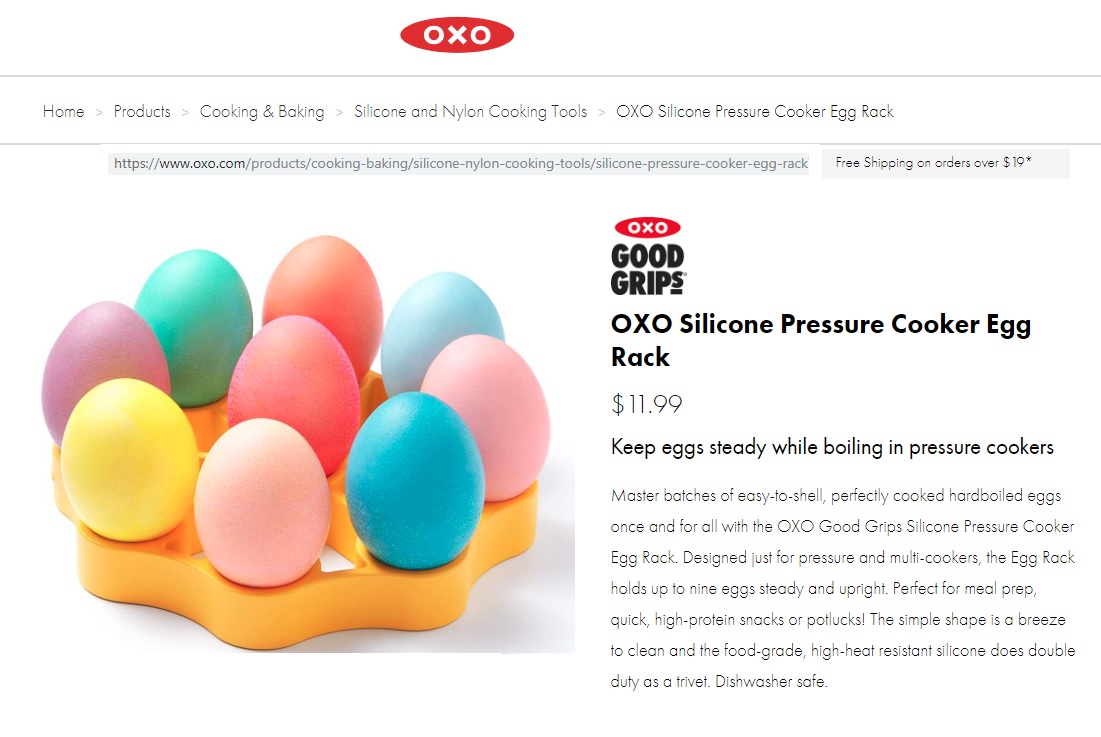The image is an online advertisement for the "OXO Good Grips Silicone Pressure Cooker Egg Rack." At the top of the ad, a prominent red oval with the brand name "OXO" in white letters draws attention. Below, there's a navigation bar featuring clickable categories such as "Home," "Products," and "Cooking and Baking."

On the left side of the image, an orange, flower-shaped egg holder is displayed. Designed to hold eggs in a circular arrangement, this egg rack has a central slot and multiple surrounding slots. It holds vibrantly colored eggs reminiscent of Easter, including shades of yellow, purple, pink, and blue.

On the right side, there is a concise product description: "OXO Good Grips Silicone Pressure Cooker Egg Rack - $11.99," highlighting its primary function to "keep eggs steady while boiling in pressure cookers." Beneath this, additional text provides more detailed information about the product's features and benefits.